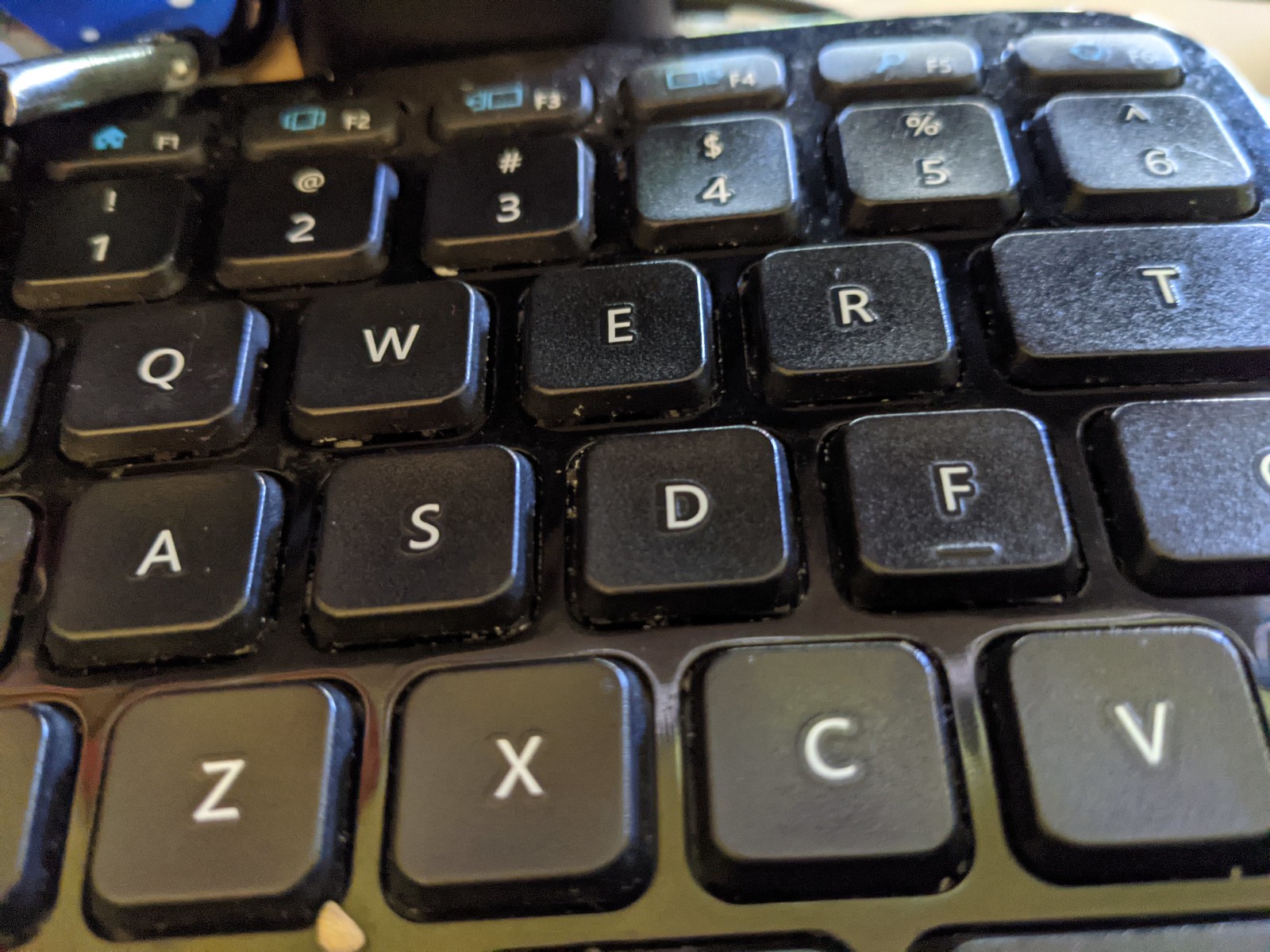This is a detailed close-up image of the left-hand section of a black computer keyboard, featuring the letters Q, W, E, R, T, A, S, D, F, Z, X, C, and V, along with the numbers 1 through 6 and the function keys F1 through F6. The keys appear to be well-worn, with signs of dust and a chip visible, suggesting it is an older or heavily used keyboard. The design looks heavier and less sleek than modern keyboards, and the presence of a rounded corner near the number 6 and F6 keys hints that it might be a split keyboard. The background of the image is indistinct.